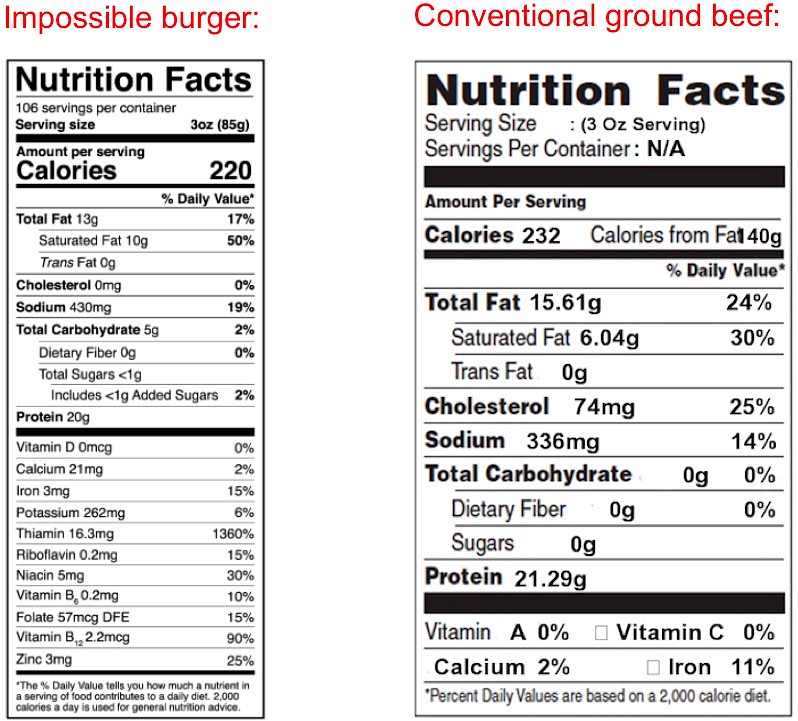This image features two distinct nutrition fact labels side-by-side for comparison. The label on the left, which is long and narrow, is topped with red text reading "Impossible Burger." In contrast, the label on the right, shorter and wider, is labeled in red text as "Conventional Ground Beef." Each nutrition label is segmented into various categories such as fat, cholesterol, sodium, vitamins, iron, and potassium, divided by thick black lines for clarity. Both labels include a leftmost column listing these nutritional items and a right column displaying their corresponding percentages. The design of the labels emphasizes the structured presentation of nutritional information, facilitating an easy comparison between the plant-based and beef options.